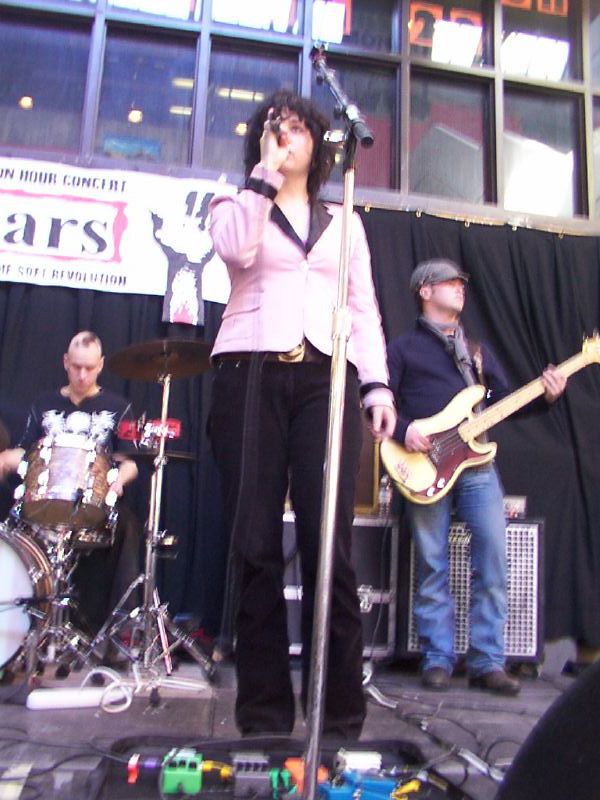The photograph captures the dynamic energy of a live concert from a fan's perspective, looking up at the stage. In the center, the androgynous lead singer stands gripping a handheld microphone, their thick, curly black hair cascading down as they wear a light pink sports blazer with a black collar, buttoned closed, and paired with black pants secured by a brown belt with a prominent gold buckle. The scene is bustling with musical equipment at their feet, including a variety of pedals and connectors in green, gray, white, orange, and blue, presumably for vocal effects and distortion.

To the back left, the drummer, who appears almost hidden behind a large silver drum set, wears a black t-shirt adorned with a white skull design. His head is shaved, leaving an odd squiggle of hair, giving his appearance a slightly eccentric flair. On the back right stands the guitarist, dressed in a blue long-sleeved shirt, a scarf, blue jeans, and boots. An unusual cap, too short to be a traditional baseball cap, sits atop his head, while he plays a yellow guitar with a rustic wood finish.

The stage is framed by a black curtain upon which hangs a sign, partially obscured, displaying the last three letters "A-R-S" and a segment of text below that suggests "Soft Revolution." Above the musicians, double rows of small window panes let in the light, implying an outdoor venue or one with significant natural lighting. The image, slightly out of focus, adds a raw, almost surreal quality to the captured moment.